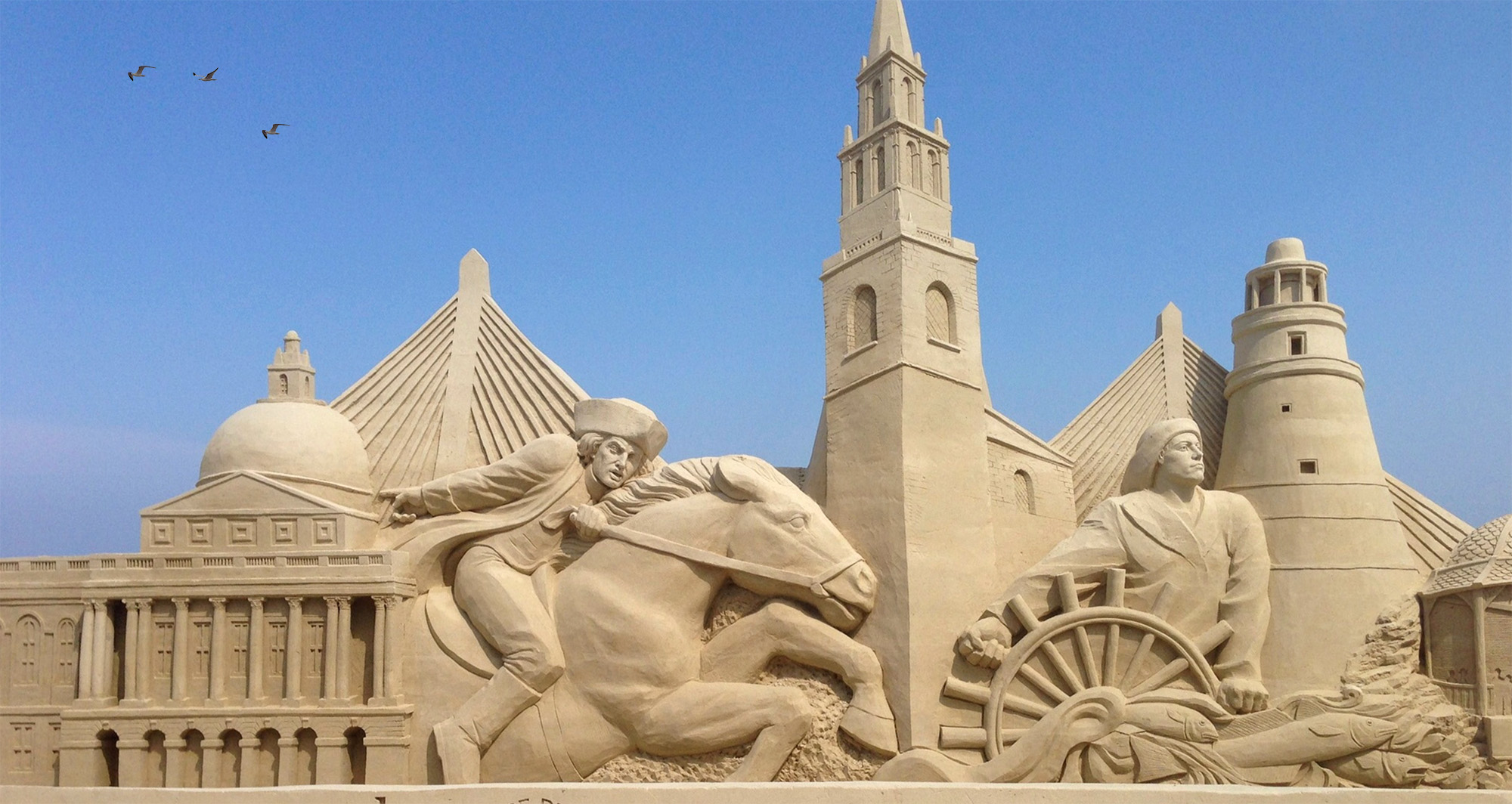The image captures a meticulously crafted and detailed sculpture of a city scene, seemingly made from a tan or brown clay-like material, or perhaps sandstone. Central to this composition is a figure resembling Paul Revere on horseback, holding a sword, evocative of historical engravings. Adjacent to this figure, a character that might be a pirate is navigating with a ship's wheel. Surrounding these central figures are various architectural elements, including a large cathedral-like building, a structure resembling the U.S. Capitol, a lighthouse, and a smaller building. A triangle-shaped monument and details such as fish are also intricately etched into the sculpture. In the upper left corner of the image, three birds soar high against a bright blue sky, adding a sense of depth and liveliness to the scene. Overall, this photograph captures a highly detailed and artful depiction of historical and nautical themes set against a serene sky.